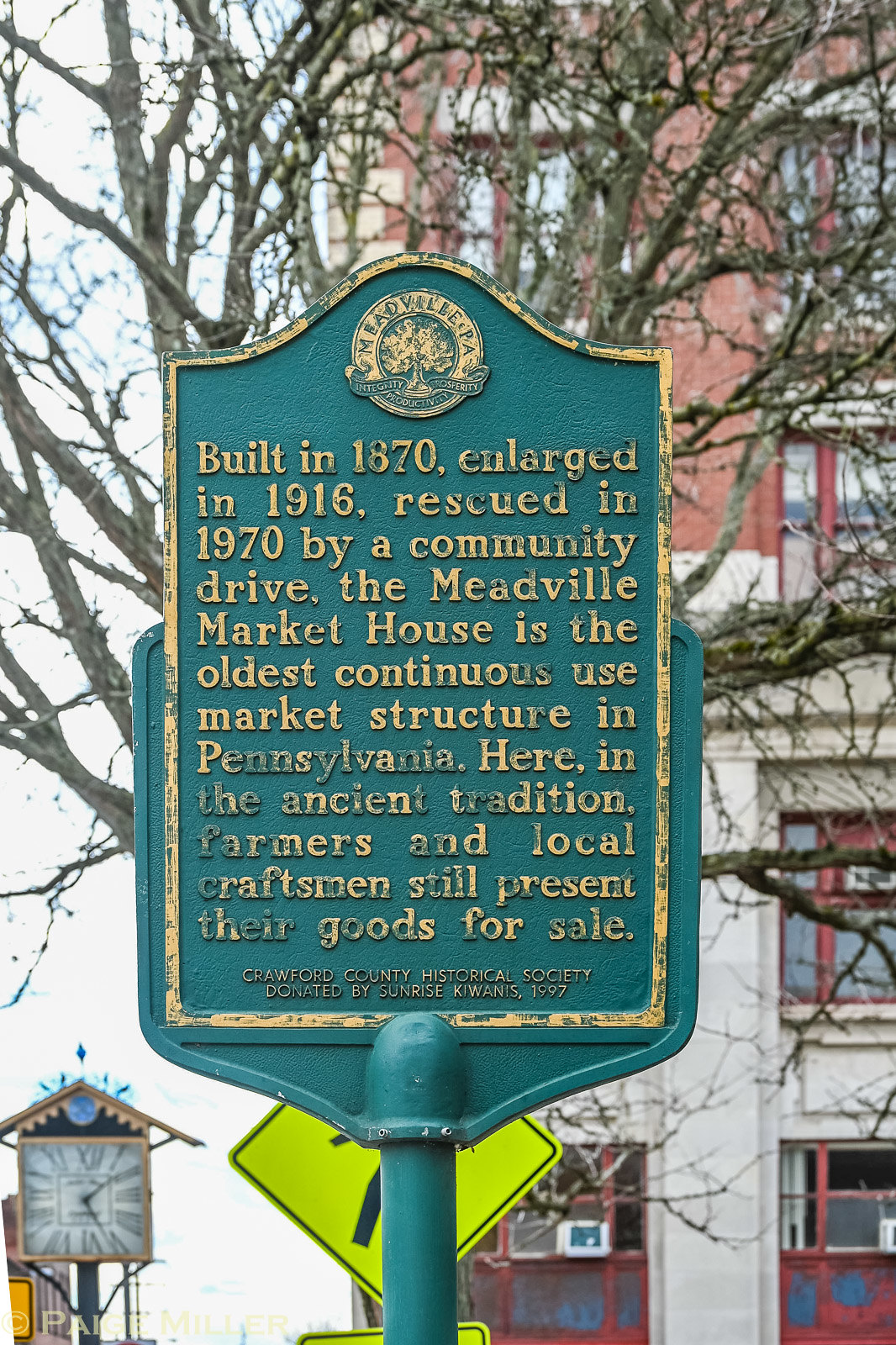This outdoor daytime photograph captures an old metal sign, likely made from a worn, turquoise-blue painted material, which has faded over time. The top of the sign features an arched design, reminiscent of a hill, with a gold circle that has similarly faded. The sign is framed by gold trim with inscriptions in raised print. At the very top of the sign, it reads "Meadville, PA." Below this, the inscription details: "Built in 1870, enlarged in 1916, rescued in 1970 by a community drive. The Meadville Market House is the oldest continuous-use market structure in Pennsylvania. Here in the ancient tradition, farmers and local craftsmen still present their goods for sale." At the bottom, in smaller raised print, it states "Crawford County Historical Society, donated by Sunrise Kiwanis, 1997."

The sign is mounted on a matching turquoise-blue metal pole. In the background, barren branches of a tree stretch across the scene, and a white sky looms overhead. To the right, a brick building is partially visible. Additionally, in the lower left corner, there appears to be a square clock with a slanted roof, indicating the time around 1:26. This detailed image evokes a sense of heritage and historical continuity amidst a timeless landscape.